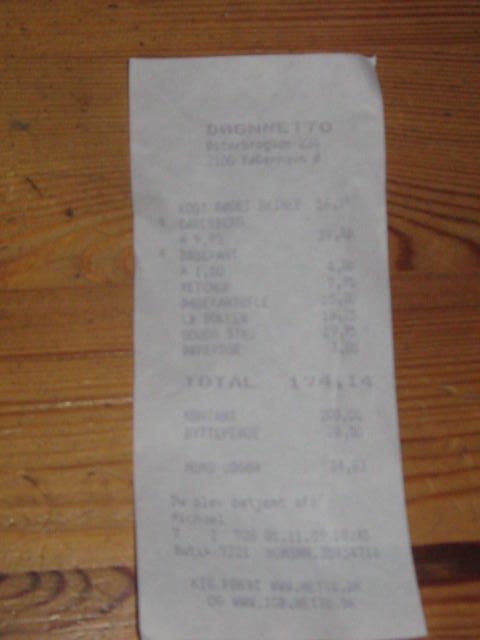A faded receipt lies on a wooden hardwood floor. The receipt, worn and indistinct, reveals only its total amount of $74.14 in somewhat legible print, as the rest of the details, such as the items ordered or the store name, remain obscured by the faded print. The wooden floor beneath the receipt features noticeable grains and knots, showing off its natural patterns and darker variations. Scuff marks and black streaks add character to the well-used flooring, suggesting a history of frequent use.